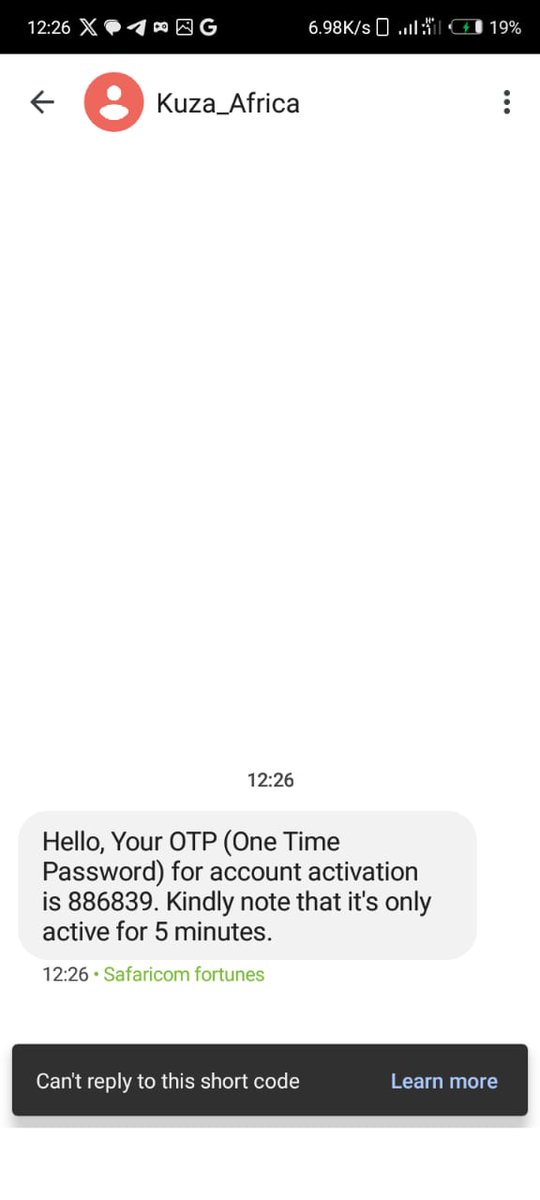This detailed caption describes a screenshot taken from an Android device, showcasing a Google text chat or a messaging app. The screenshot captures a message exchange, specifically an OTP verification text from "Kooza_Africa." The solitary message, timestamped at 12:26, reads: "Hello, your OTP one-time password for account activation is 886.839. Kindly note that it's only active for five minutes." Below this message, the text "Safari Calm Fortunes" is visible. The screenshot also displays an application notice with the message "can't reply to this short code" and a link labeled "learn more."

At the top of the image, a black status bar indicates the time as 12:26 and includes several icons: the X (formerly known as Twitter) icon, a chat icon, a paper airplane icon, a gaming icon, a photo icon, and the Google 'G' logo. The status bar also shows the data transfer rate "6.98 K per second," followed by icons representing a phone, signal strength, battery energy, and the battery level at 19%.